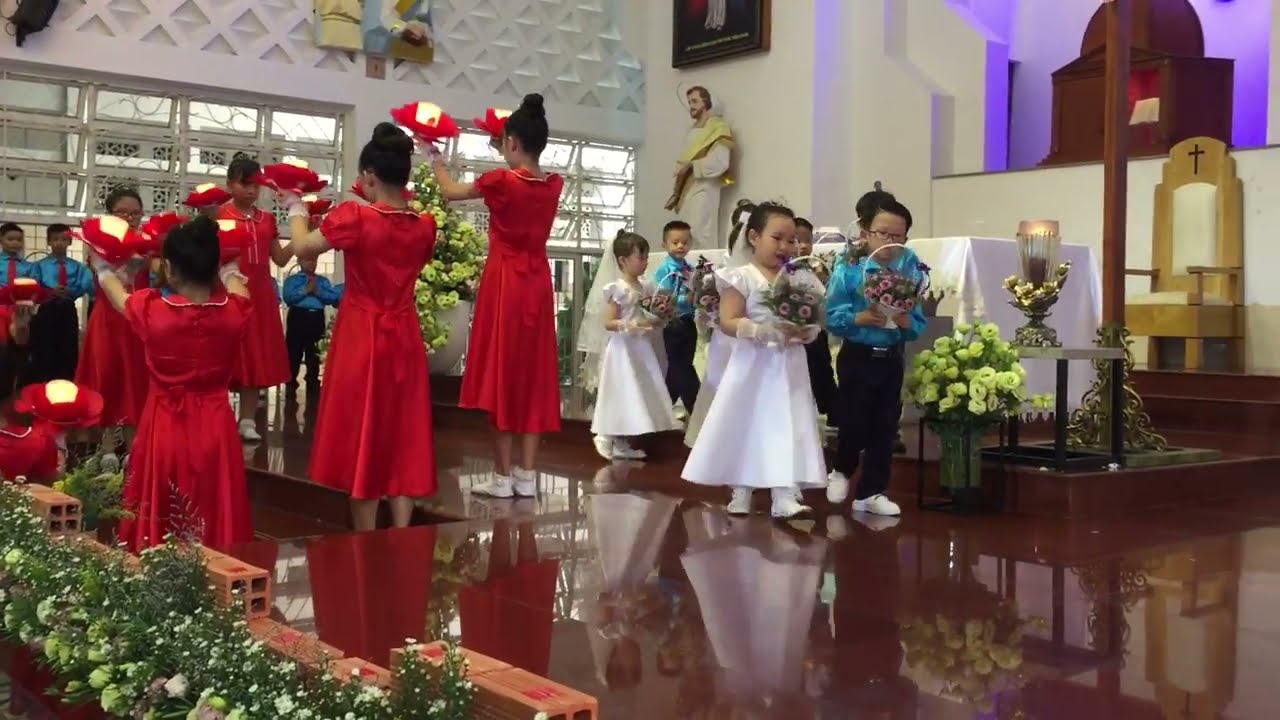The photograph captures a vibrant and meticulously arranged ceremony, likely of a religious nature, featuring two rows of about a dozen young Chinese girls. Each girl is adorned in a red dress and white shoes, holding bouquets of flowers and candles in both hands. One row has its back to the camera while the other row faces them, forming a picturesque walkway up a set of wooden stairs that leads to a stage. The scene is set in what appears to be a church, evidenced by the wooden pews filled with spectators, some of whom are engaged in taking photos and videos to document the event. The stage is flanked by a line of little boys in blue button-up shirts and black pants, emphasizing the coordinated and ceremonial nature of the occasion. The background features church architecture, including an archway to the center left and glass panes to the right, adding a serene and spiritual atmosphere to the entire scene.